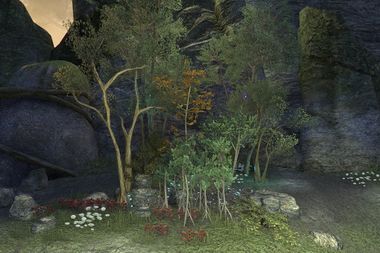This image is a detailed scene of a dimly lit, nighttime outdoor area featuring a small cluster of trees and various plant life. In the background, imposing gray stone formations rise, covered sporadically in green moss. The stones are punctuated by a large boulder to the side, and the setting sun or a low-set moonlight peeks through a crack among the rocks at the top left, casting a muted glow over the landscape.

The trees in the foreground vary in height, from short to medium-sized, suggesting a mix of young and slightly older growths. Some roots are exposed, adding to the rugged feel of this natural enclave. Below the trees, the ground is adorned with an array of small bushes and flowers. Yellow-flowered bushes sit behind clusters of green bushes, and to the very left, little patches of white and red flowers dot the grassy field, adding subtle splashes of color.

At the heart of the composition, slightly left of center, stands a dead tree with bare branches, providing a stark brown contrast against the predominately gray and dark-hued environment. The possibility of a small creek running through the scene adds an element of intrigue, though it's vague and not clearly defined. The overall scene is rich with natural textures and subdued hues, creating a deep, contemplative atmosphere.